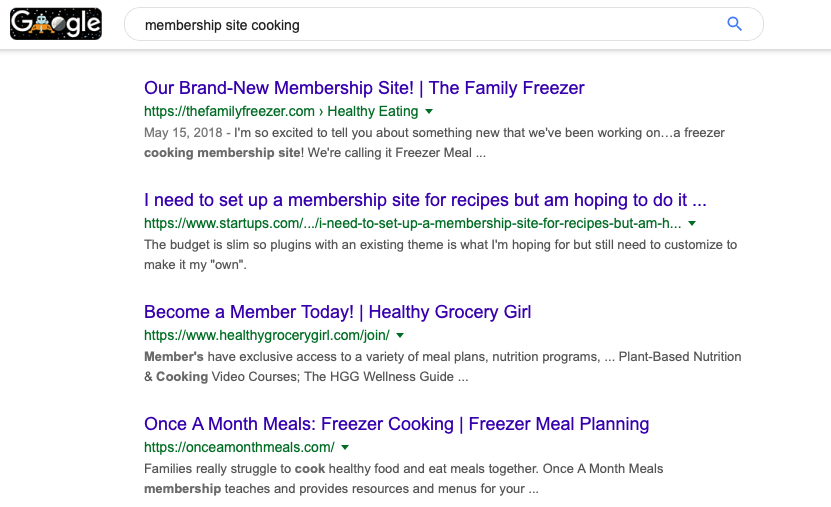The Google Membership Site Cooking page features a recent Google Doodle themed around space exploration, with the second "O" in "Google" depicted as a moon and the first "O" as a lunar lander. The page includes four prominent links:

1. **Our Brand New Membership Site, The Family Freezer**: Accompanied by excited text introducing a new Freezer Cooking Membership Site.
2. **Startups.com**: Discusses setting up a new membership site for recipes, noting budget constraints and the use of existing themes and plugins.
3. **Healthy Grocery Girl**: Invites users to become members and gain exclusive access to a variety of meal plans and other resources.
4. **Once a Month Meals**: A membership program focusing on freezer cooking, aimed at families struggling to cook healthy meals and eat together. It provides teaching and resources for effective meal planning.

The page has a clean layout with a white background, blue links, and black text.